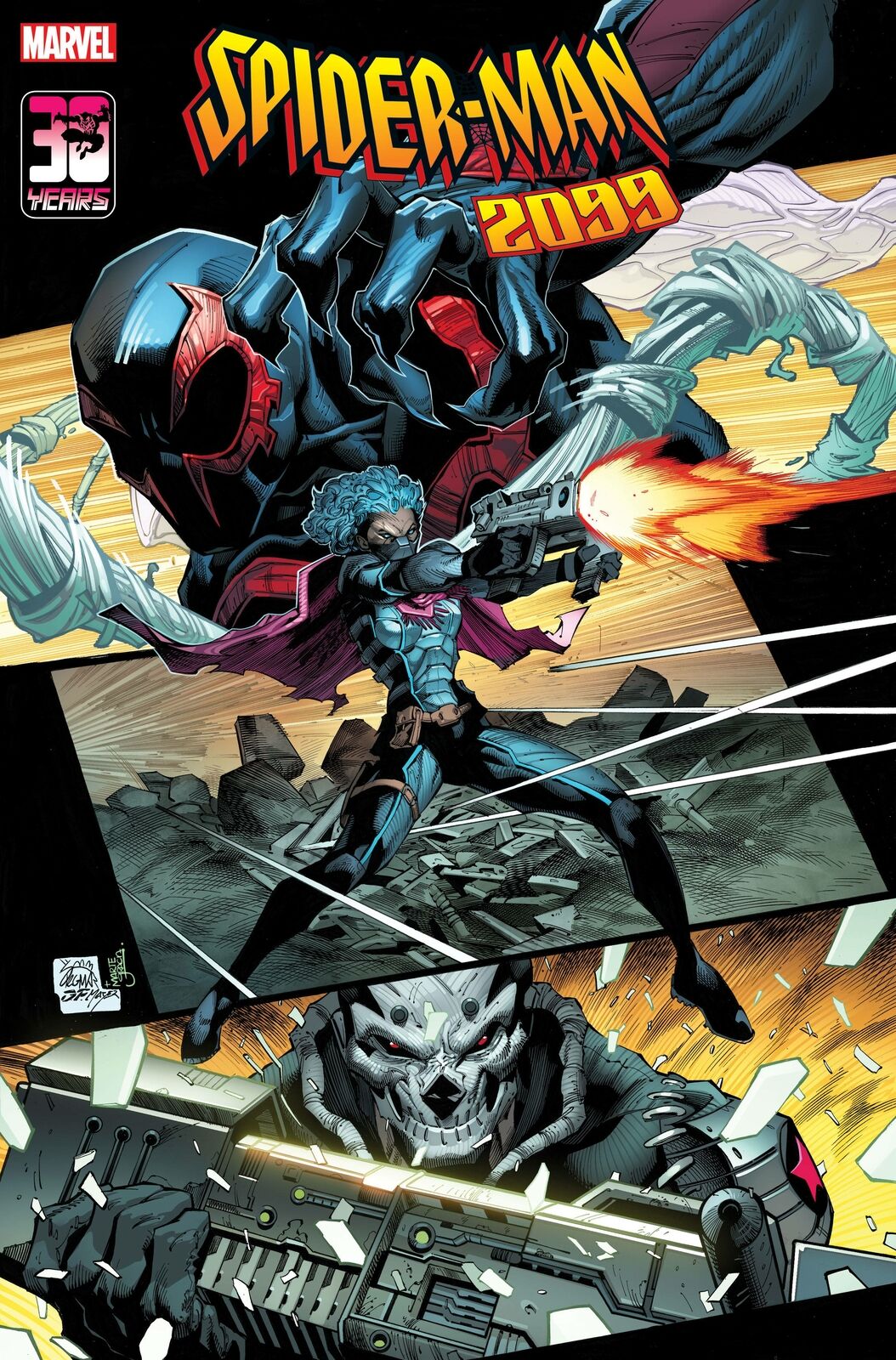This is a detailed comic book cover for Marvel's "Spider-Man 2099," featuring vibrant, animated artwork. In the top left corner, white text over a red background reads "Marvel," accompanied by a "30 Years" logo. The title "Spider-Man 2099" is displayed prominently in a bold, spiky font with yellow, black, and red colors. The cover is divided into three distinct sections, each showcasing a different character. At the top, Spider-Man is depicted in a futuristic suit with red and blue colors, differing from the traditional Spider-Man look. The middle section features a woman wearing a mask and armor, wielding a flame gun; she has a striking purple cape. At the bottom, another menacing figure with a skull head holds a formidable weapon. The entire cover is richly illustrated, promising an adventurous journey into a futuristic Spider-Man storyline.